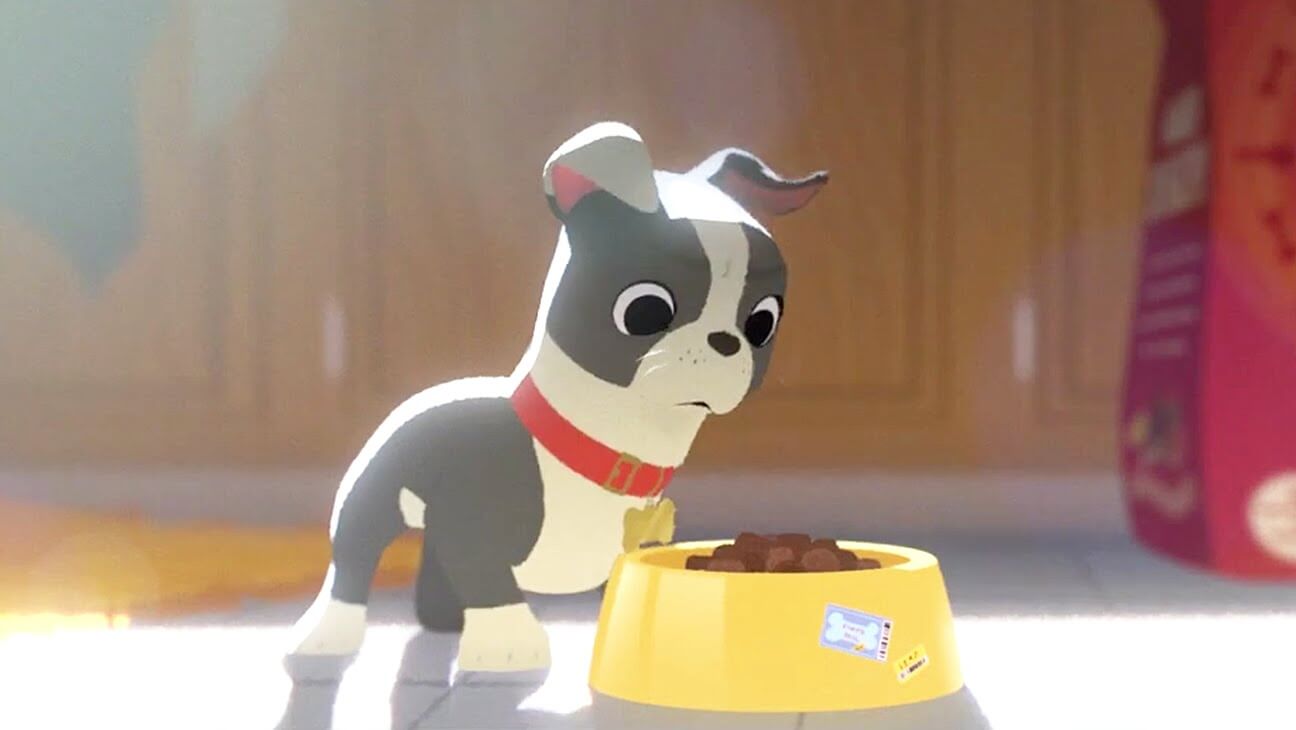This animated image portrays a small, grey, and white dog, possibly a pug, with floppy ears and a distinctive fur pattern. The dog's face, chest, and legs are white, while its back, around its eyes, cheeks, and parts of its ears are grey. It has black eyes, a black nose, and a red collar around its neck with small whiskers poking out. The pink inner parts of its ears are visible. The dog is intently staring at a yellow food bowl in front of it, which contains brown dog food. The bowl features a purple sticker with a white bone design and another yellow price sticker. Behind the dog, to the right, there is a red bag of dog food with indistinct lettering. The background shows brown cabinets stretching across the scene, a white tiled floor, and an orange rug situated to the left of the image.